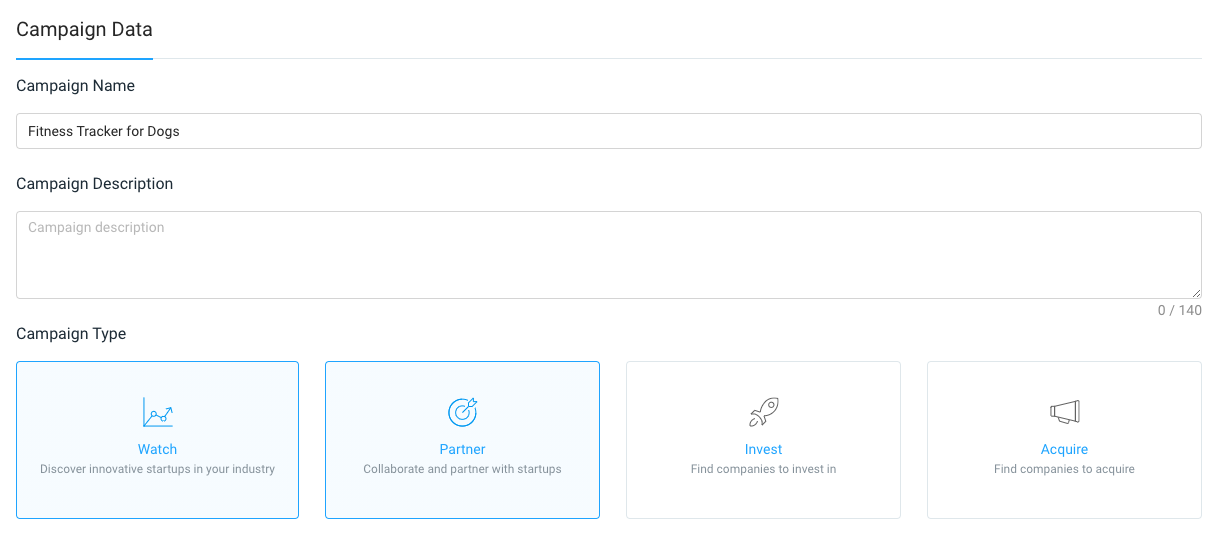This image is a screenshot of a form page designed for inputting campaign data. At the top left corner, the page header reads "Campaign Data." Below it, a label states "Campaign Name," followed by an input field populated with the text "Fitness Tracker for Dogs." Beneath the "Campaign Description" label, there is another text box with the placeholder text "Campaign Description" in gray, indicating that it is awaiting input. Further down, the label "Campaign Type" appears, accompanied by options or entries labeled as "Watch" and "Partner."